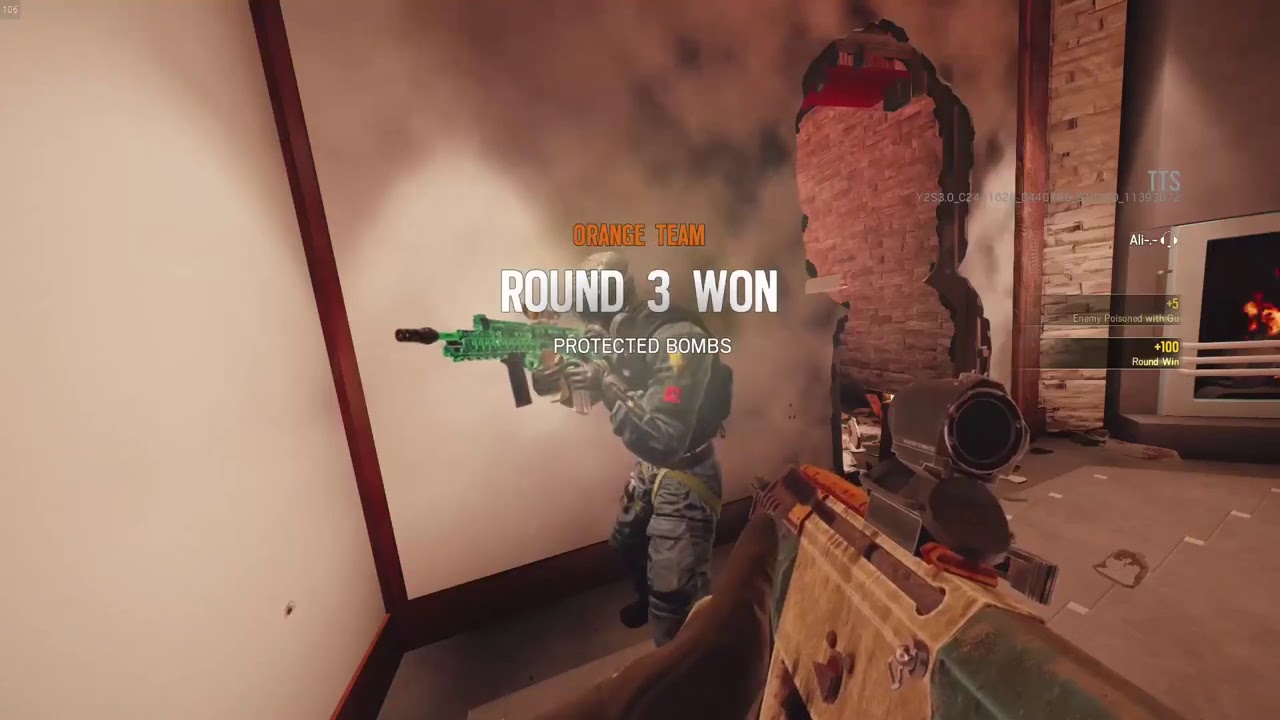The screenshot captures a first-person shooter video game where the player is part of the Orange Team during "Round 3-1" with the objective "Protected Bombs." The in-game HUD displays various scores like "+5" and "+100," along with a label "TTS" at the top. Dominating the foreground is the player's character holding a scoped weapon with their left hand, aimed at an opposing soldier wearing gray military fatigues with yellow accents, a red patch, and a helmet. The enemy soldier wields a green gun and is positioned towards the left side of the screen. The background features a white wall with brown borders, a large hole revealing a brick wall beyond, smoke, and a fireplace insert on the far right. The setting is filled with a predominant color scheme of brown, green, a little orange, and off-white, contributing to the detailed and immersive combat environment.